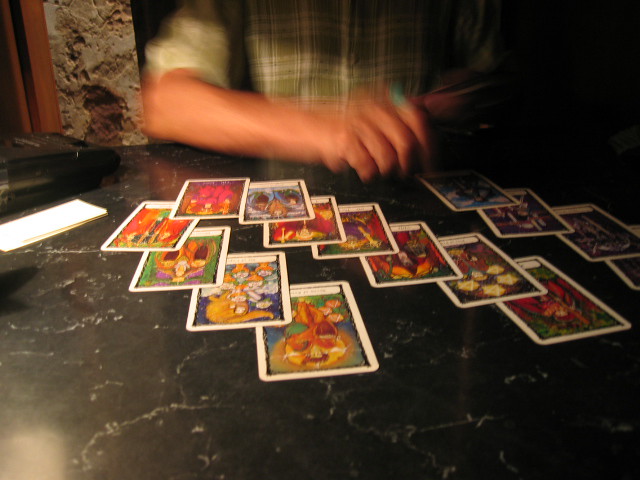The image features a Caucasian man engaging in a tarot card reading, set against a striking backdrop of black stone with white veins. The man is dressed in a green plaid shirt and is captured in motion, his hand reaching towards a card in a swirl formation. The cards boast a vibrant array of colors—yellows, oranges, blues, purples, reds, and whites—with each card showcasing a colorful image and words at the bottom, though not completely legible. Near his hand, a card with yellow and orange hues stands out, while a blue and white card is visible behind his left arm. Other colorful cards are positioned around him: a purple card to his left, a blue card beneath his arm, and a red card nearby. A black box is placed in the top left corner of the image, further adding to the scene's intriguing elements. This action shot captures the dynamic moment of divination amidst a visually compelling array of colors and textures.